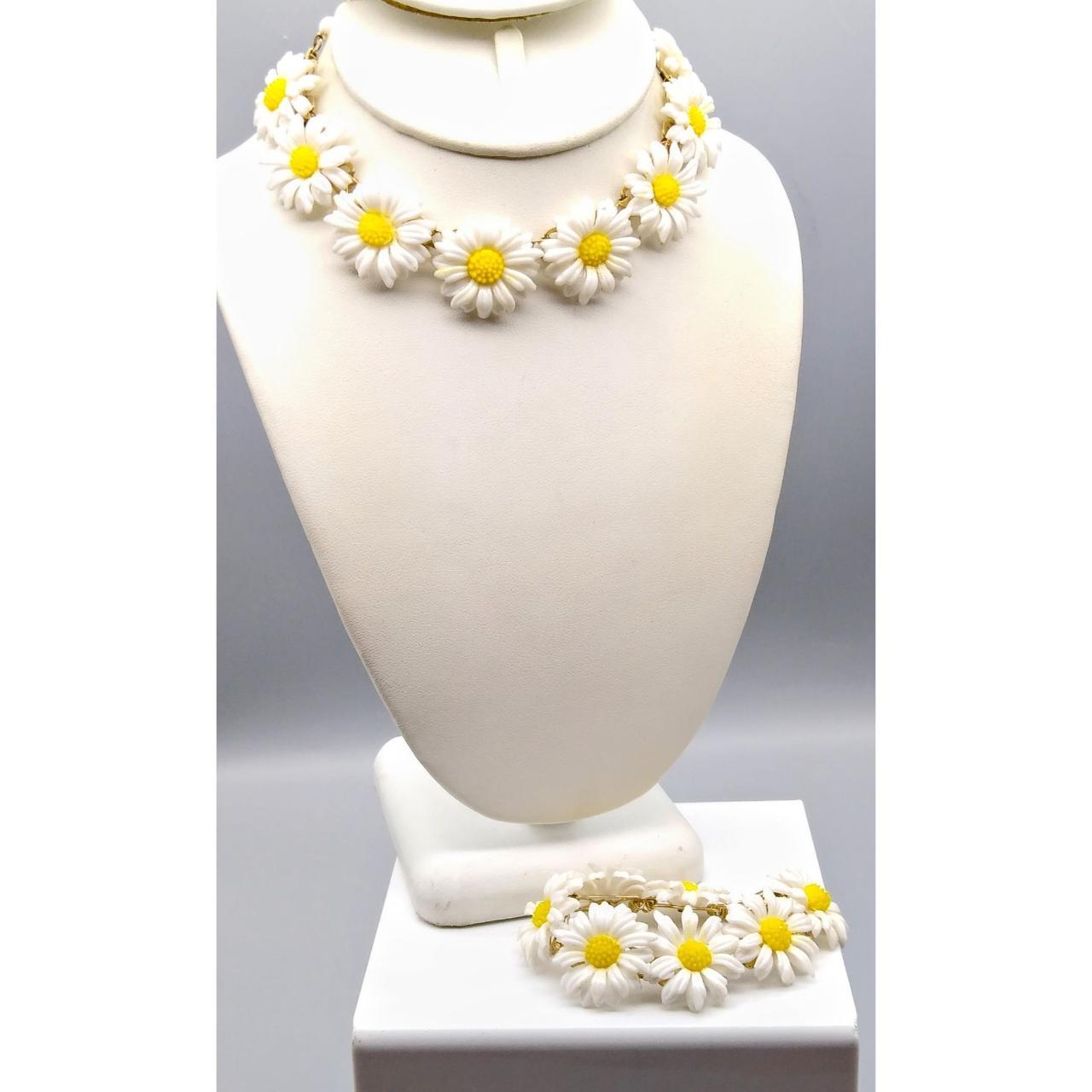The image showcases a sleek jewelry display against a subtle gray background. Central to the composition is a headless, white mannequin stand set on a pedestal of a slightly off-white, cream color. Adorning the mannequin is a delicate necklace crafted from white petal flowers with yellow centers, reminiscent of daisies or chamomile. In front of the mannequin, matching jewelry, potentially a bracelet, is carefully laid out on the white base. The background transitions into a soft, uniform gray, enhanced by gentle shadowing and lighting effects, lending a minimalistic yet elegant feel to the image. At the very top, there is a faint glimpse of what might be an attachment for the head part of the mannequin. This photograph, likely a stock image, expertly highlights the floral-themed jewelry in a clean, refined setting ideal for display purposes.